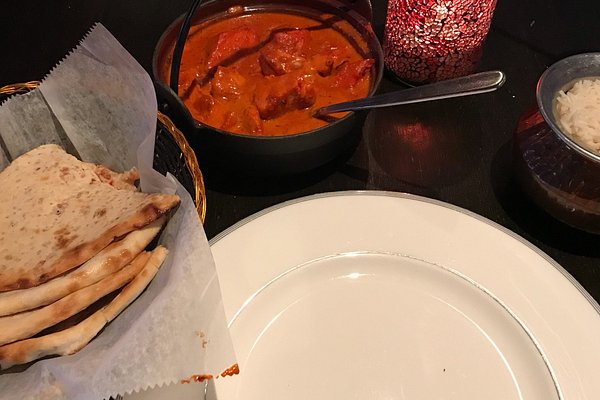The image depicts a casual dinner scene on a brown wooden table, capturing a mix of diverse elements in an amateur, unarranged manner. Central to the image is an empty white ceramic plate, hinting at a meal that has yet to be served. To the left, a gold basket lined with white paper holds pieces of naan, some pulled apart or ripped in half. Adjacent to the plate lies a small aluminum bowl filled with white rice. Towards the top of the image is a black pot or bowl containing what seems to be a red sauce, likely tikka masala, with large chunks of meat submerged in it. A large silver serving spoon is visible, adding to the informal dining setup. Above and slightly to the right, a red, intricately designed candle holder emits a warm glow, casting light across the scene. The overall setting exudes a spontaneous, homey atmosphere, with a variety of foods and utensils haphazardly placed, suggesting a ready-to-eat meal captured just before serving.